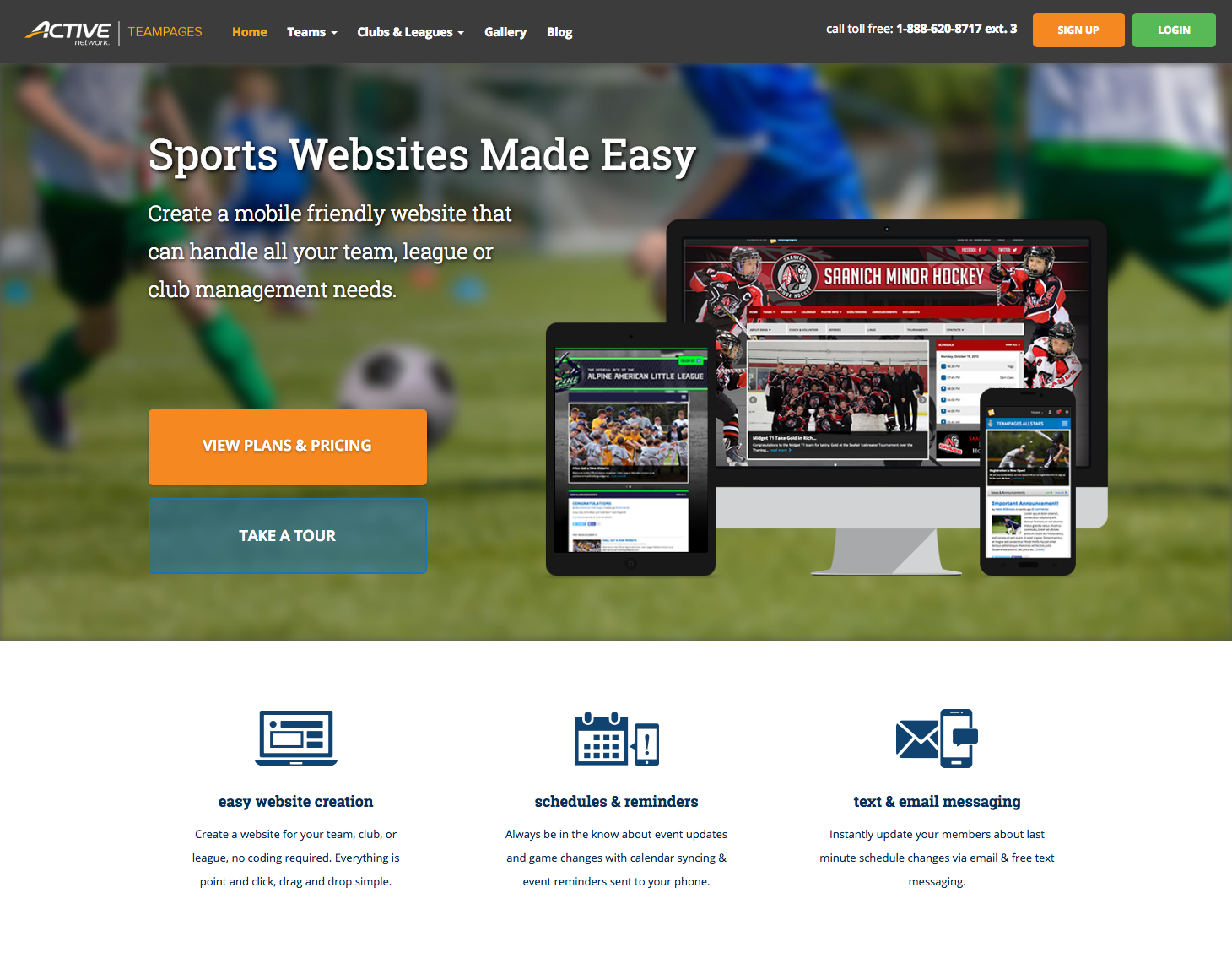The upper left corner of the image features the words "Network" and "Team." Moving across the top navigation bar, there are menu options labeled "Home," "Teams" with a dropdown menu, "Clubs" and "Leagues" with top-down menus, "Gallery," and "Blog." On the right side of the navigation bar, there is a toll-free number: 1-888-620-8717, extension 3. Adjacent to the contact number, there is an orange "Sign Up" button and a green "Login" button, both featuring white font. The navigation bar is set against a dark gray strip.

Below the navigation bar, a background photograph encompasses the main promotional text, which reads: "Sports Websites Made Easy. Create a mobile-friendly website that can handle all your teams, leagues, or club management needs." Positioned on the left side below the promotional text are two buttons: an orange "View Plans and Pricing" button and a semi-transparent teal "Take a Tour" button, both with white font.

To the right of the text, there is an image of a monitor displaying the website, with a tablet and a cell phone placed in front of it, showcasing responsiveness across devices.

At the bottom of the image, set against a white background, are three icons in a row, each with descriptive text underneath:
1. "Easy Web Creation" - Create a website for your team, club, or league. No coding required. Everything is point-and-click, drag-and-drop simple.
2. "Schedule and Reminders" - Always be able to...